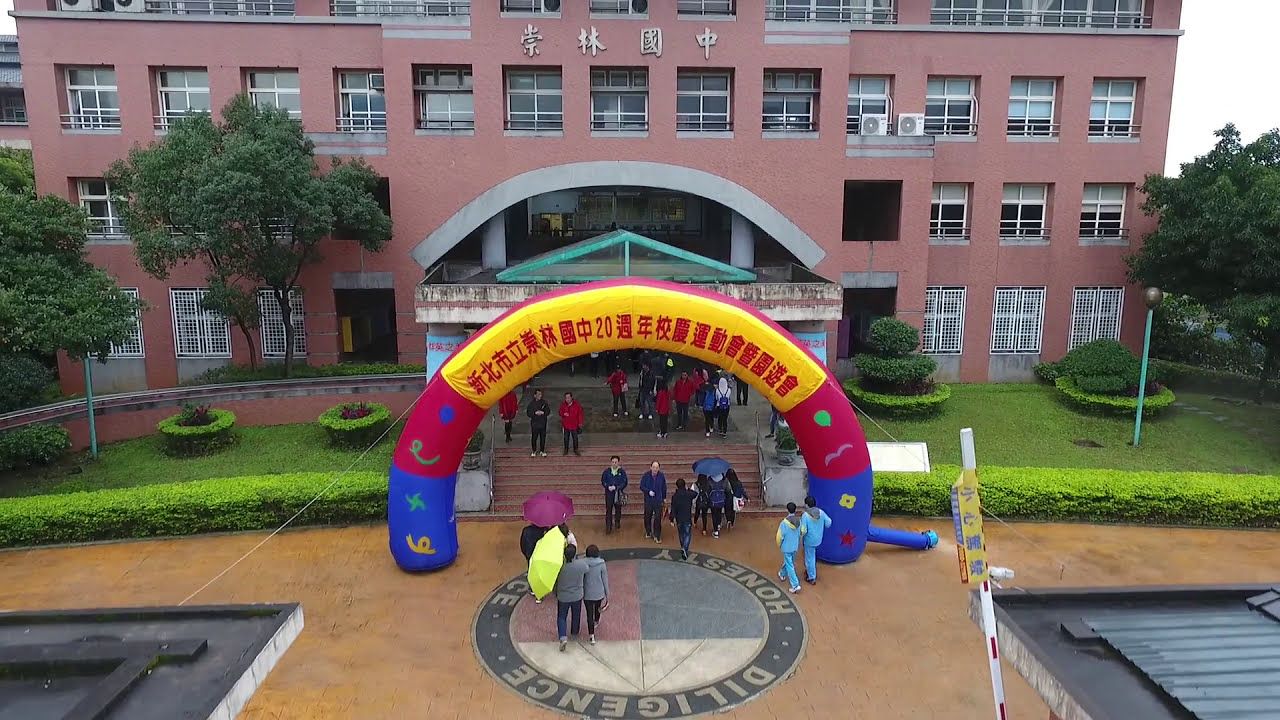This is a horizontal rectangular aerial image of a large red-brick building, likely a school. The building, characterized by numerous windows, features an arching concrete entranceway accompanied by a decorative area. Leading up to the entrance are about five steps. Prominently displayed in front of the entrance is an inflatable arch, with the top section colored yellow and the sides transitioning into red and blue. The yellow section of the arch bears Chinese characters. The surrounding environment includes patches of grass, bushes, and trees, adding a touch of green to the scene. The area in front of the steps is a concrete courtyard, within which a large circular feature is at the center. Several people are visible walking in and out of the building, many holding umbrellas, indicating rainy conditions. The sky above is overcast, contributing to the overall dreary, wet atmosphere.